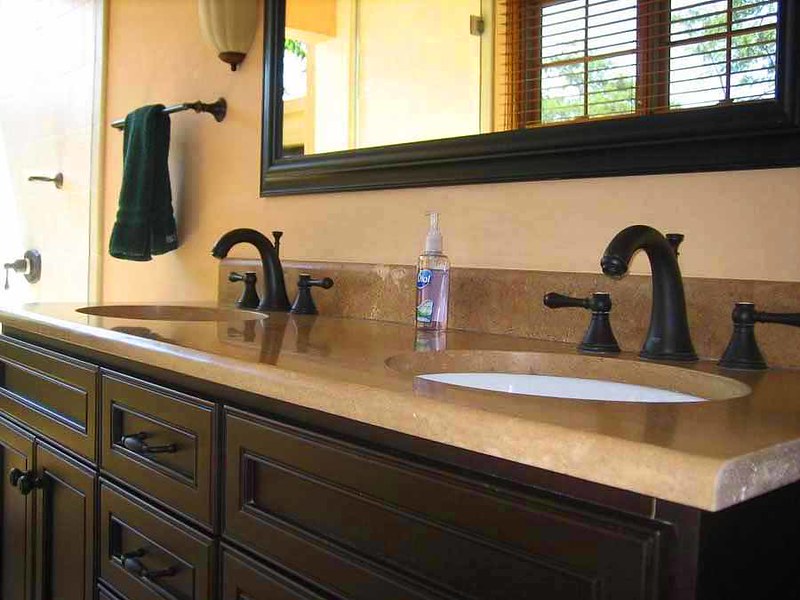The image showcases a section of a well-designed bathroom. The walls are a soft pinkish-beige color, providing a warm backdrop. A white door with a silver handle and a small hook is visible. Dominating the scene is a large, elegant mirror with a dark wood frame, reflecting a double window, part of another window above a door, and a white cabinet. 

The vanity area is striking, featuring a dark wood finish with significant storage space: large drawers on the right, smaller drawers in the center, and cabinets on the left. Two oval-shaped sinks with stylish black faucets and turn knobs are set into a beige and white mingled countertop. 

The countertop holds a clear bottle of Dial liquid soap with a blue label and pump top. A towel holder, possibly bronze or gold, holds a green towel, adding a touch of color. A small light fixture with a bronze base and a white shade illuminates the area. The overall aesthetic of the bathroom is both functional and visually appealing.